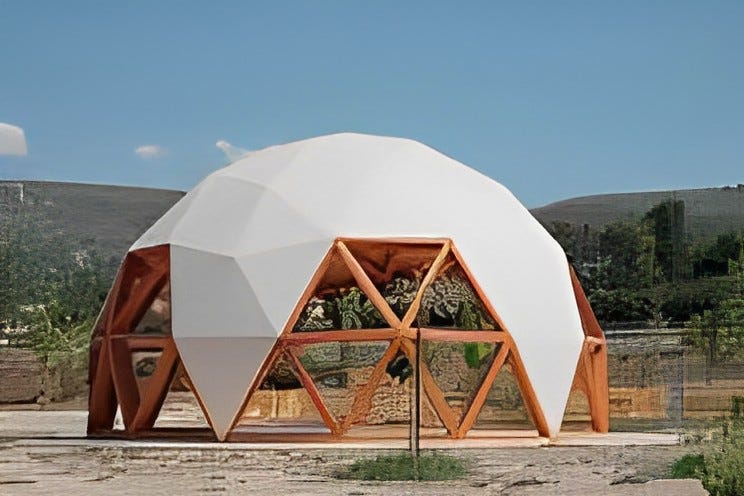This image captures a striking daytime scene featuring a geometric dome structure set against a picturesque blue sky. The dome, approximately 25 feet high, is constructed from light golden-brown wood formed into hexagonal and triangular patterns, creating a grid-like appearance. The dome's cover is partially white, interspaced with open sections that offer glimpses through its framework. Situated on sandy, dirt-covered ground interspersed with patches of grass, the dome is enclosed by a fence. The background showcases a range of brown hills or mountains dotted with small plants and trees, enhancing the natural beauty of the setting. This modern architectural installation resembles a tent or canopy and is devoid of any interior elements or occupants, accentuating its open and airy design.